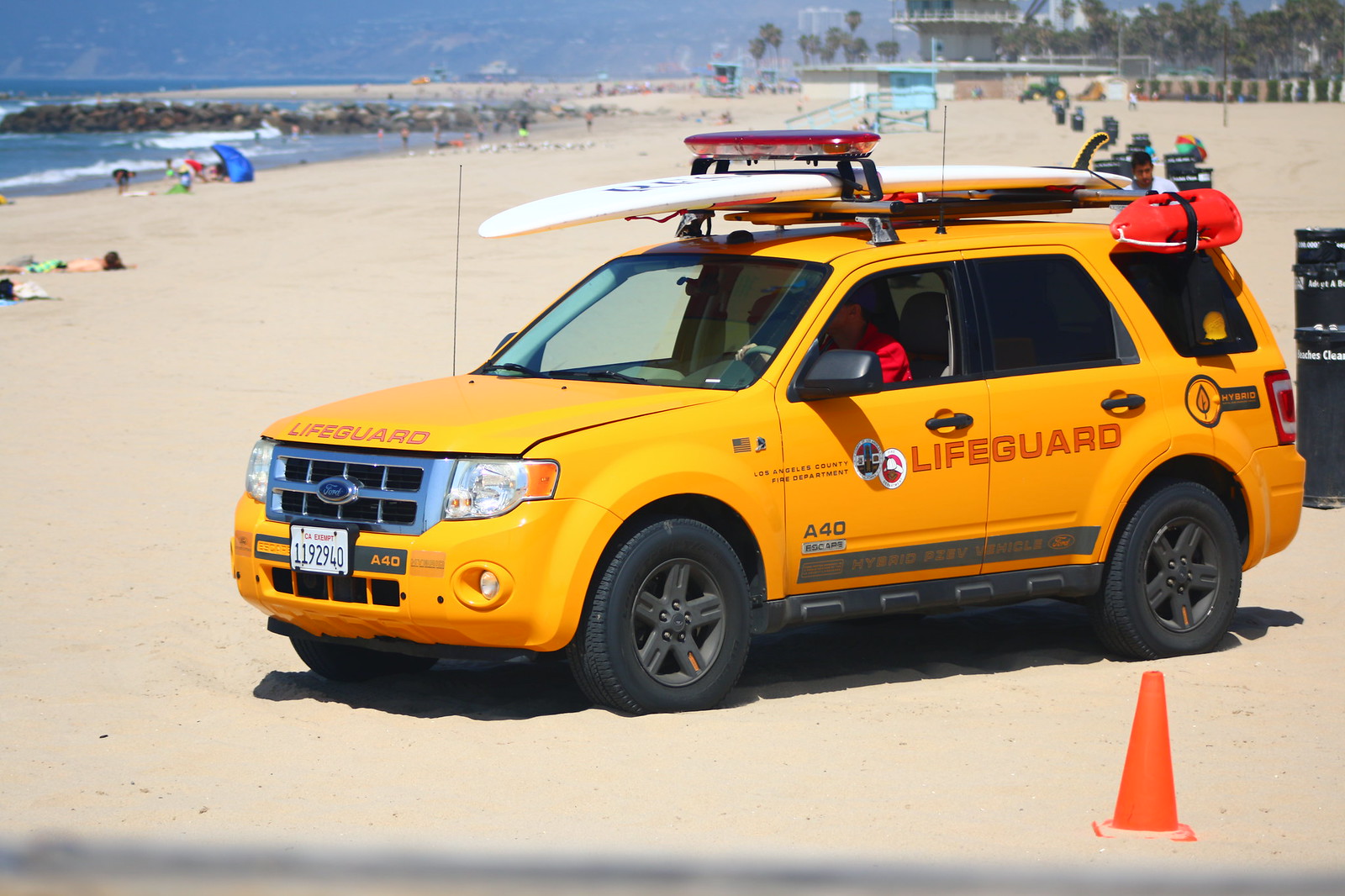This image captures a vibrant scene at a seaside beach dominated by a yellow Ford SUV emblazoned with "Lifeguard" on its side. The vehicle, identifiable by its grille with the Ford emblem and the license plate number 1192940, is turned slightly to the left. The SUV, a hybrid model indicated by the A40 hybrid PIEV vehicle marking, features prominent black tires, side view mirrors, and visible front bumper and taillights. Inside, a driver in a red jacket operates the left-hand drive vehicle. Atop the SUV sits a roof rack secured with a surfboard and various lifeguard safety equipment including red beaming lights, life jackets, and a life preserver. The foreground of the image is composed of smooth sand scattered with an orange safety cone nearby. The beach is bustling with activity; people lounge on towels, stroll, and engage in various activities. The backdrop features glimpses of the blue sea, a clear sky, and distant buildings interspersed with trees. The overall scene gives a vivid portrayal of the beach environment enriched with essential lifeguard apparatus, ensuring safety and vigilance.